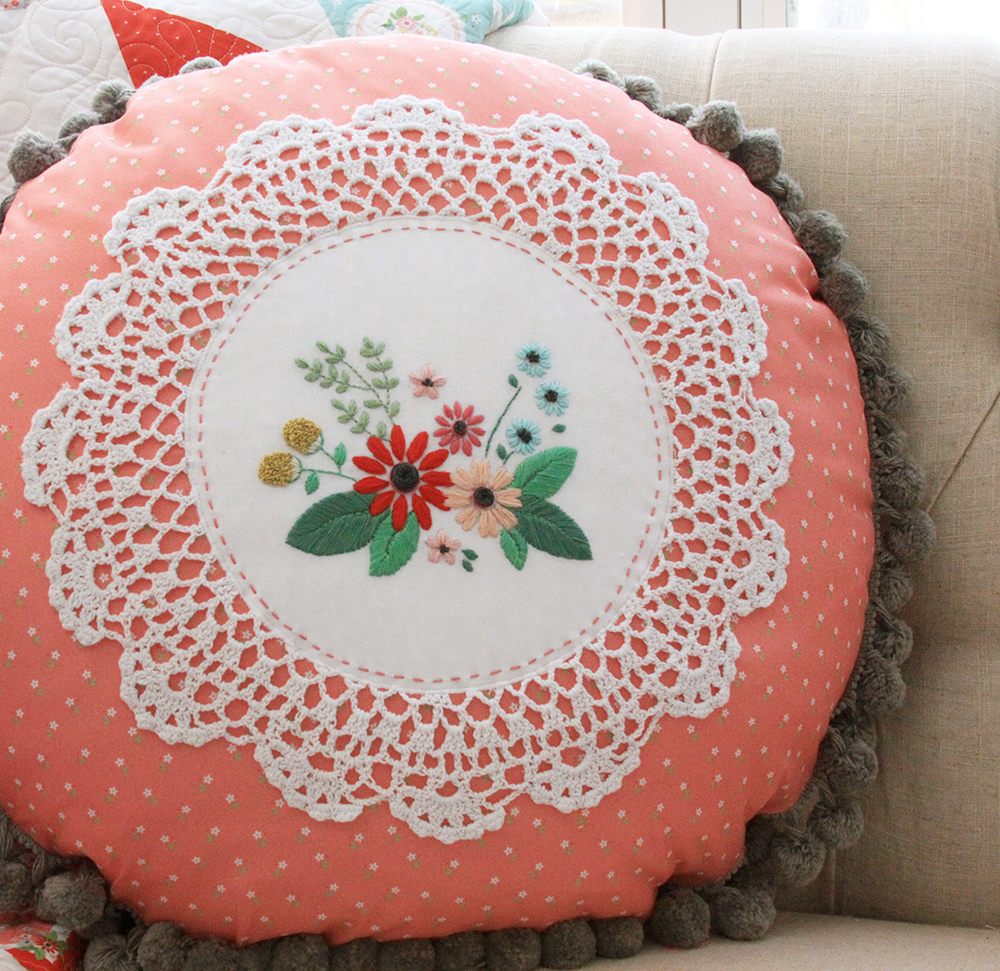The photograph features a strikingly detailed coral-colored circular pillow that dominates the composition. Placed atop a grey sofa cushion, the pillow's vibrant coral hue creates a vivid contrast with the neutral background. At the center of the pillow, intricate woollen work encircles a patchwork centerpiece, noticeable for its delicate white base. 

This patchwork showcases an exquisite embroidery pattern, depicting a cluster of flowers and leaves. The embroidery is a flourish of colors, boasting flowers in shades of red, pink, light pink, blue, and yellow, alongside green leaves. The surrounding area of the pillow is adorned with a subtle small flower print, complementing the central design. 

Adding further texture, the pillow is bordered with a charming woolen pattern. In the top left corner of the photograph, a portion of a multicolored quilt peeks into the frame, adding an additional layer of warmth and coziness to the scene.